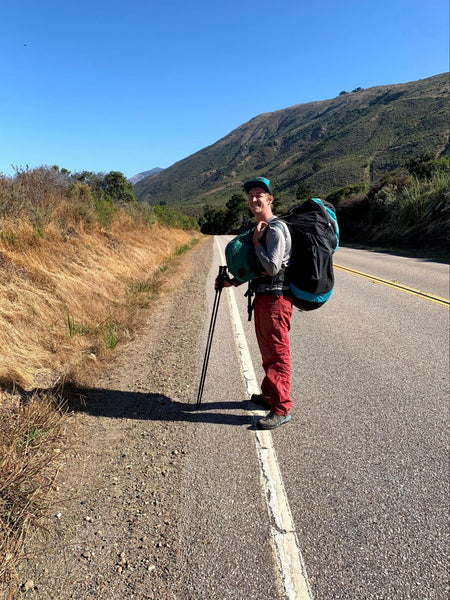A man stands on the white fog line along a double yellow-line two-lane highway, facing away from the road and towards tall, rolling hills. He is equipped with extensive backpacking gear, including a large black and light blue backpack strapped to his back and a smaller light blue sack wrapped around his chest. His hand grips both walking sticks in one hand while the other hand rests under a pack strap on his shoulder. He is dressed in a gray long-sleeved shirt, red pants, and hiking boots, topped off with a black and green baseball cap. The scene is set under a sunny sky with banks lining each side of the road, obscuring the view beyond them. On his left, the grass appears yellow and dead, while ahead, a tall mountain looms with patches of green vegetation and visible roads winding through the trees. The man appears to be in mid-hike or possibly hitchhiking, posing for the photograph with the picturesque backdrop unfolding behind him.